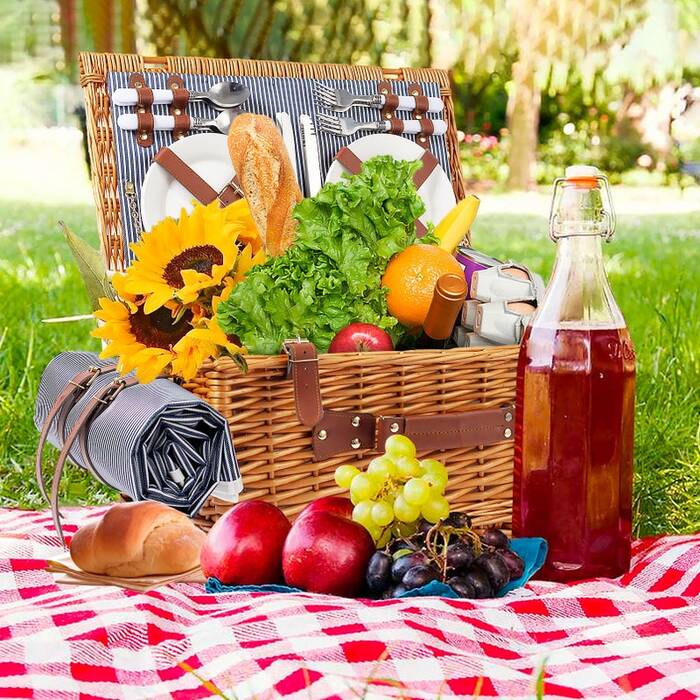This photograph captures a picturesque picnic scene set on a verdant lawn. Central to the image is a rectangular brown wicker picnic basket with a leather handle and straps, positioned atop a red and white striped cloth. The basket is open, revealing neatly strapped utensils—knives, spoons, and forks, along with two plates fixed to the lid. Protruding from the basket, we see an assortment of items: large Romaine lettuce heads, a bottle of wine, a carton of eggs, an apple, an orange, a baguette, and a pair of large sunflowers. Additionally, there's a mysterious purple box on the left side of the basket. Scattered around the cloth are a variety of fruits and items fit for the feast: clusters of both yellow and purple grapes, another three apples, and a single bread roll. A bottle of iced tea with a cork top, holding an amber-red liquid, adds a final touch to this detailed and colorful picnic arrangement.